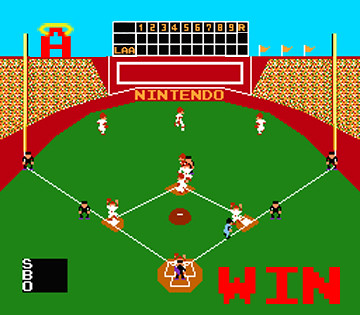This image is a screenshot from a vintage Nintendo baseball video game. Dominating the upper portion is a stadium with a blue sky backdrop. On the left side of the scoreboard is a prominent red "A" with a yellow halo, signifying the LA Angels. The scoreboard itself is black and features three vertical rectangles, with only the bottom one labeled "LAA." To the right of the "A," the scoreboard shows inning numbers from 1 to 9, followed by "R," but no scores are posted. Just right of the scoreboard, three orange pennant flags wave above a red stadium filled with spectators represented by a yellow abstract pattern. Below the scoreboard, the outfield wall is red with "Nintendo" written in yellow at the center.

The outfield is a vast expanse of green grass, where three players in white uniforms with red hats are positioned. There are five umpires in total: one at the outfield line, two at first and third bases, and one behind home plate, all dressed in black shirts, black hats, and blue pants. In the lower right corner of the image, "WIN" is displayed in large red letters. The bottom left corner features a black box with white letters "S," "B," and "O" aligned vertically.